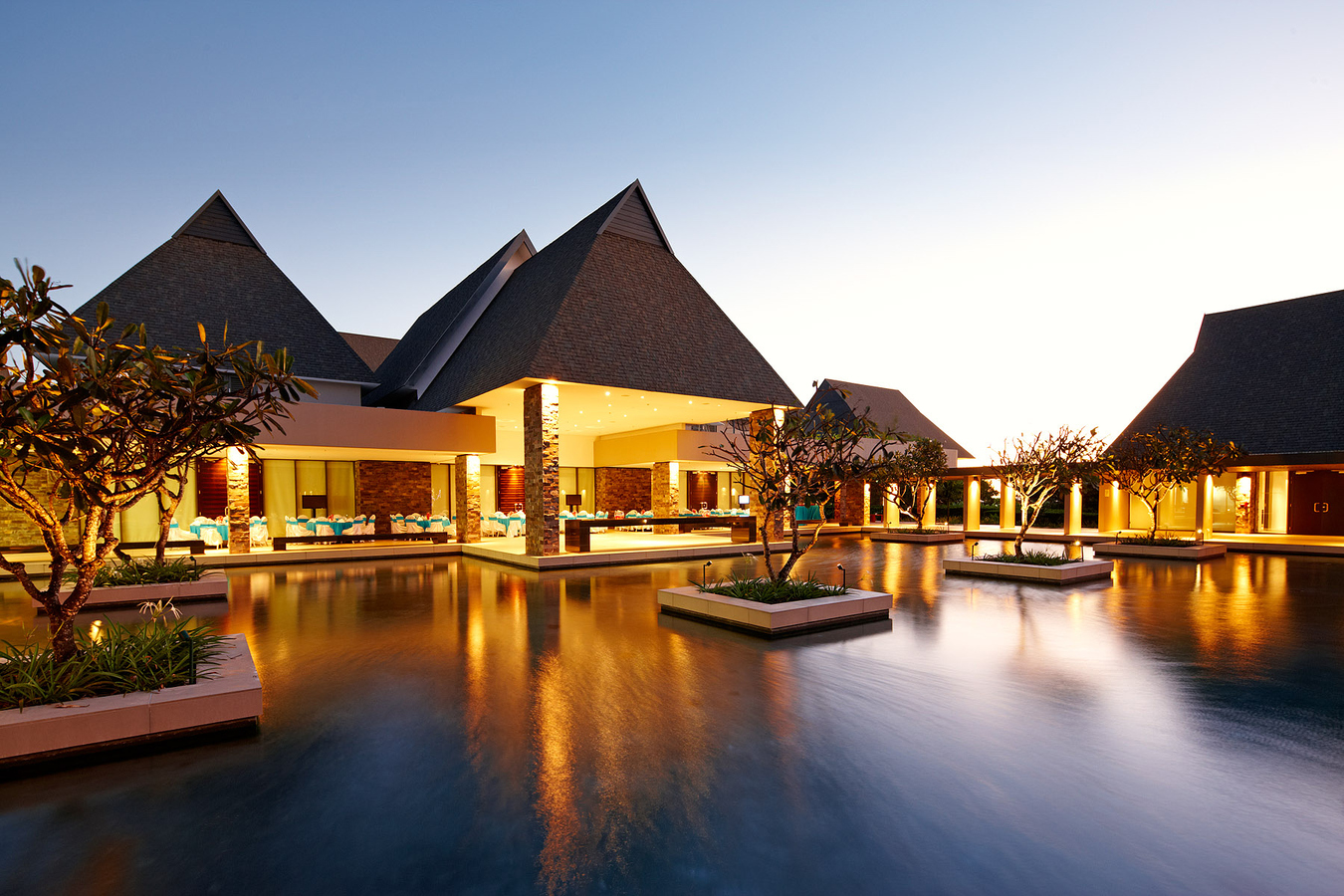The image showcases a serene, horizontally aligned rectangular scene, likely set in the early evening or nighttime. Dominating the foreground is a large, calm, rectangular body of reflective, brownish-gray water interspersed with four square concrete planters, each housing a small tree. This tranquil setting sits in front of what appears to be a large, two-story luxury house or resort, featuring multiple sections with brown, triangular-tipped roofs. The well-lit building extends across the middle of the image, from left to right, and its back porch is bathed in a warm yellow glow from numerous lights. This illumination highlights an arrangement of white and blue chairs at various tables, suggesting an outdoor dining area. The scene is further accented by a long walkway that meanders around the water, inviting visitors to explore the picturesque setting. The sky transitions from a clear blue on the left to a hazy white on the right, hinting at the fading daylight and creating a peaceful, inviting ambiance.